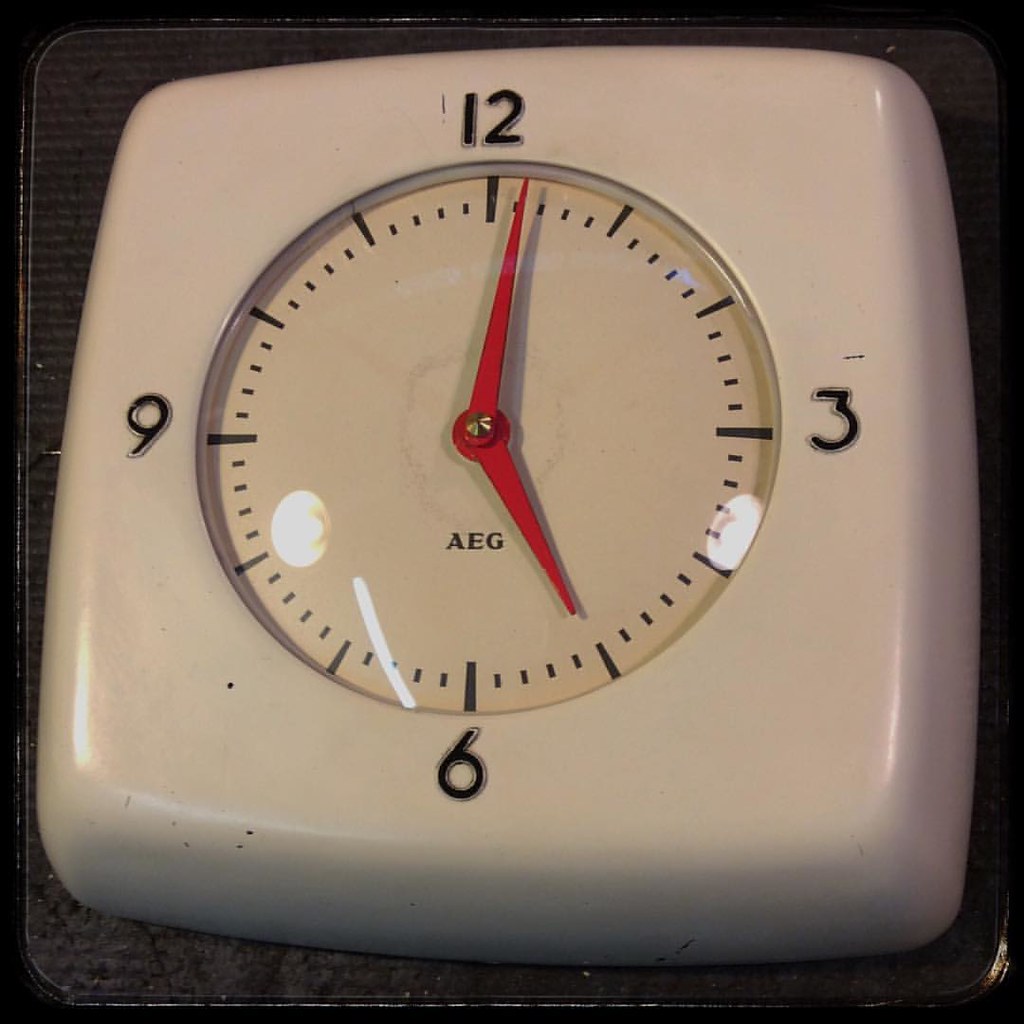This is a vintage-inspired, miniature travel clock designed to be placed on a bedside table. Crafted from a ceramic or stone-like material, the clock has a prominent design featuring only the 12, 3, 6, and 9 numerals, with the remaining hours marked by smaller lines. Minute increments are also indicated with even finer lines. The clock hands are made of red metal and are encased behind a cover that appears to be glass, though it might be a hard plastic. The manufacturer's name, A.E.G., is prominently displayed in capital letters. The clock is roughly palm-sized, square in shape with gently rounded edges, adding a touch of elegance to its vintage aesthetic.